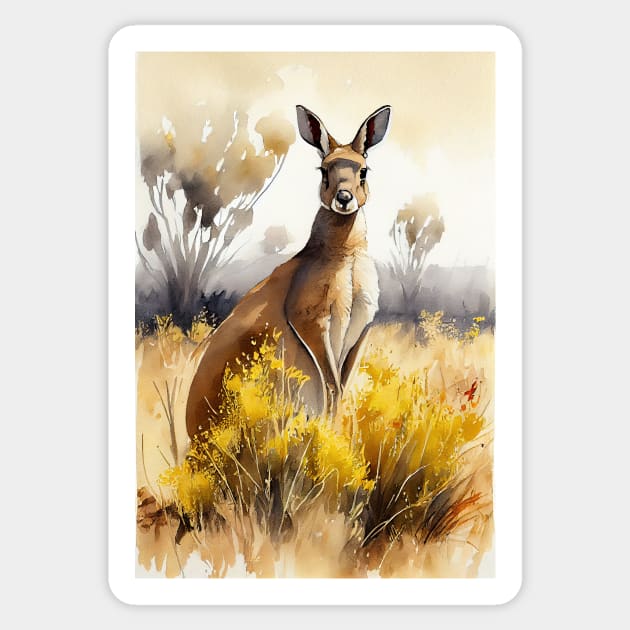This image is a watercolor painting of a light brown kangaroo standing upright on its back legs, looking directly at the viewer with large, perked-up ears. The kangaroo's chest is a lighter, almost white color. Its front legs are partially obscured by yellow shrubs in the foreground. The background consists of a vast, dry prairie with brown grass, a few scattered reddish plants, and some distant trees. The sky is a light blue, almost white, creating a soft, unfocused backdrop. The scene is surrounded by a white frame, enhancing the prominence of the kangaroo as the central focus of the painting.